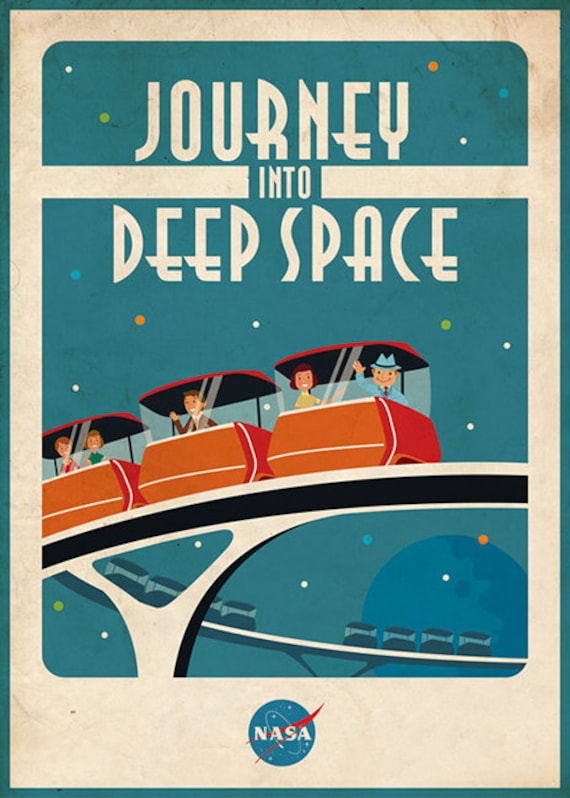The image is a detailed, vintage color poster with a cartoon-like illustration, reminiscent of the 1950s to 1960s era. The poster has a dark aqua border, enclosing a cream-colored background. At the top, a dark blue background showcases the large, centered title "JOURNEY INTO DEEP SPACE" in white capital letters, spaced out over three lines. White lines underline "Journey" and "Deep Space," with additional lines framing the word "Into" horizontally. Small star-like speckles in orange and white dot the blue background, adding a cosmic feel.

Dominating the center of the poster is an illustration of a monorail, depicted with a large black and white curved track supported by white beams. Three orange tram cars ride the track, each with glass windows. Inside the cars, people can be seen smiling and waving, conveying a sense of joy and adventure.

At the bottom of the poster, the iconic NASA logo is prominently displayed. The logo is dark aqua with "NASA" in white letters, featuring a red swash through the center and a stylized blue orbit with stars. The lower edges of the poster appear slightly yellowed, contributing to its vintage appearance.